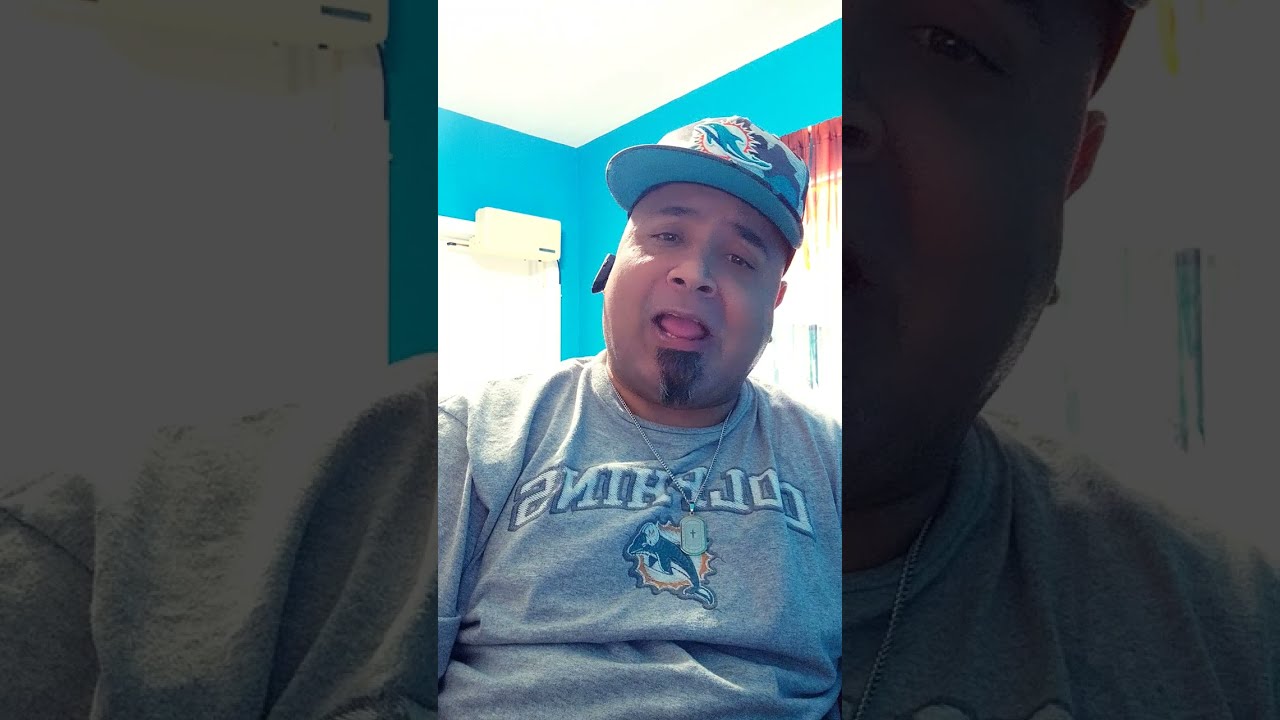The image captures a close-up of a Hispanic man engaged in a video conference call or FaceTime, viewed from the waist up. He has brown skin, a small goatee, and a visible soul patch beard. The man is mid-speech with his mouth open and tongue visible. He wears a multi-colored Miami Dolphins hat, predominantly blue with white and orange accents, and a gray t-shirt emblazoned with the Dolphins logo and the word "DOLPHINS" in white text. He also has a square metal piece on a necklace giving the impression of dog tags and an earpiece in one ear. The room around him features turquoise or light blue walls, a white ceiling, and translucent curtains in orange and white. The setting includes two windows, one on each side, giving the impression of a well-lit, casual environment. The overall scene emphasizes his Miami Dolphins fandom and his focused participation in the video call.